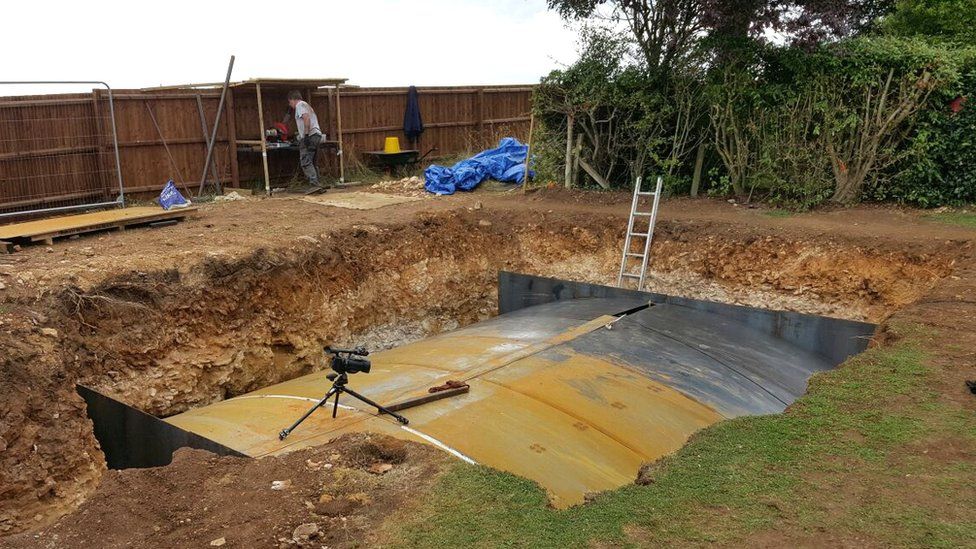In this daytime outdoor photograph, a sizable excavation site dominates the scene, surrounded by a rectangular hole approximately 12 feet deep. A large underground metal structure, appearing to be about 8-12 feet long with a gray and rust-brown hue, sits in the center of the dig. The structure rests on a gravel base, with more gravel visible around its bottom. Atop the structure, a metal ladder with six to seven rungs extends upwards, providing access in and out of the hole. Notably, both ends of the structure are lined with black pile sheet metal.

To the upper right, a man stands near a tall wooden fence, intently examining blueprints. He is dressed in dark pants and a light short-sleeved shirt, appearing to be involved in the construction work. Additional elements in the background include a small collection of trees and bushes, a blue crumpled tarp, and a sparsely grassy area around the excavation's edges. The immediate foreground and much of the surrounding area are primarily dirt, typical of a construction site, interspersed with occasional patches of grass about 10 feet from the man near the fence.